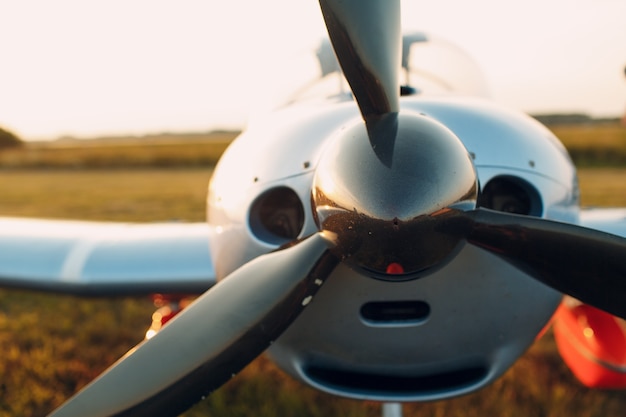This highly detailed, close-up photo vividly captures the nose of a sleek, contemporary crop-dusting airplane. Dominating the foreground, the reflective chrome propeller features three shiny blades, and the plane's immaculate polish gives off a copper-like sheen. Flanking the propeller, two circular windows resemble eyes, imparting an almost anthropomorphic appearance to the aircraft. The streamlined, smoothly curved body of the plane is accentuated by its silver wings and the cockpit's transparent glass canopy, which hints at the pilot's seat behind.

The sturdy craft appears ready for diverse terrains, equipped with flotation devices for water landings. Reddish patches in the brown field suggest it is grounded in a grassy area with a blurred, grayish backdrop providing a contrasting horizon. The forward-facing circles likely serve as headlights, and additional open vents are visible beneath the rotor. A striking red object to the right adds a splash of color, either part of the aircraft or an adjacent item. The overall impression is of a modern, meticulously designed aircraft set against a subdued landscape.